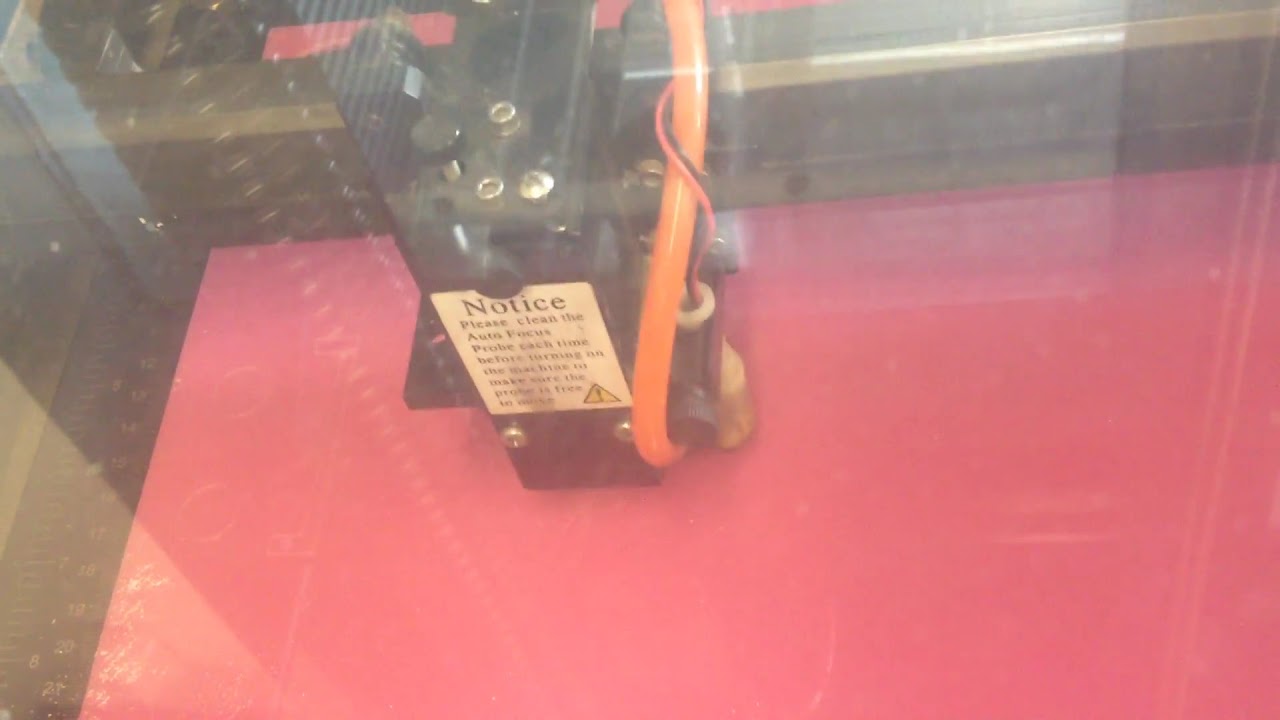In a manufacturing or production setting, an intricate mechanical device enclosed within a plexiglass case is prominently displayed. The device is a tall, rectangular, primarily black machine adorned with metal screws and a conspicuous black button. An orange wire extends from the bottom, wrapping around to the back. Accompanying this are red and black wires that also trail from the bottom, intertwining with the orange wire. A prominent feature on the device is a white sticker with black lettering that reads: "Notice, please clean the autofocus probe each time before turning on." Above this notice, there's a caution symbol—a yellow triangle with a black exclamation point. Also notable is a red surface situated behind the device, adding a vivid contrast to the scene. The entire setup is meticulously protected behind a clear glass or plexiglass enclosure.